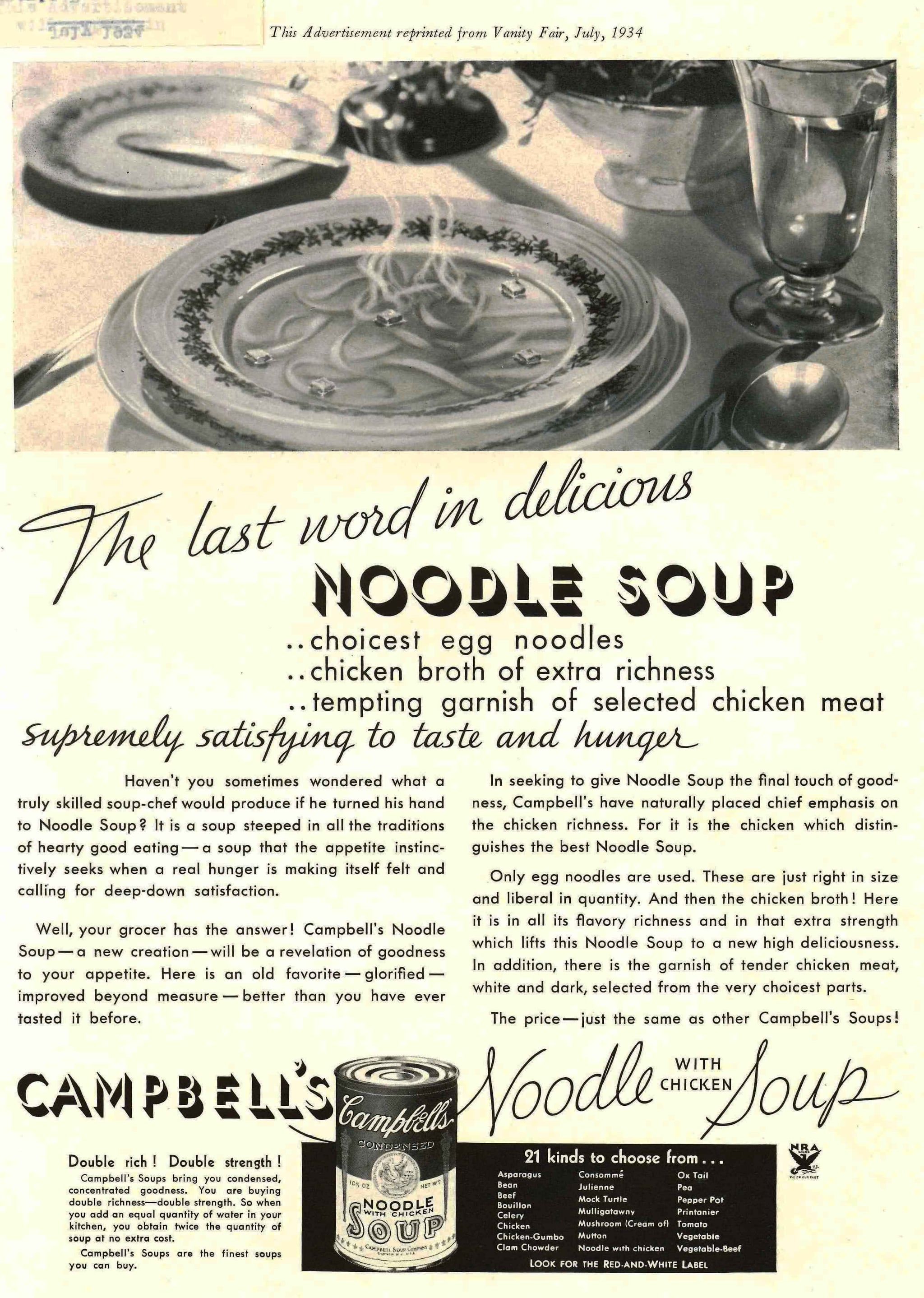This is a meticulous black-and-white advertisement for Campbell’s Noodle with Chicken Soup, reprinted from Vanity Fair, July 1934. The ad showcases a professionally set dinner table featuring a central steaming bowl of soup, likely made of ceramic or china with a gold wreath border. The elegant place setting includes a plate underneath the bowl, a spoon, and a fork, along with a water goblet and a bread and butter plate to the left. A decorative flour dish with floral or brocade elements adorns the middle of the table.

Above this setup, the ad prominently states, "This advertisement reprinted from Vanity Fair, July 1934." Below the image, the tagline reads, "The last word in delicious noodle soup," followed by three bullet points: choicest egg noodles, chicken broth of extra richness, and tempting garnish of selected chicken meat. It further emphasizes the soup's supreme satisfaction of taste and hunger. Additional text informs that the price remains the same as other Campbell’s soups. On the bottom left, a can of Campbell’s Noodle with Chicken Soup is depicted alongside a black box listing 21 kinds to choose from, offering a variety of soup options.